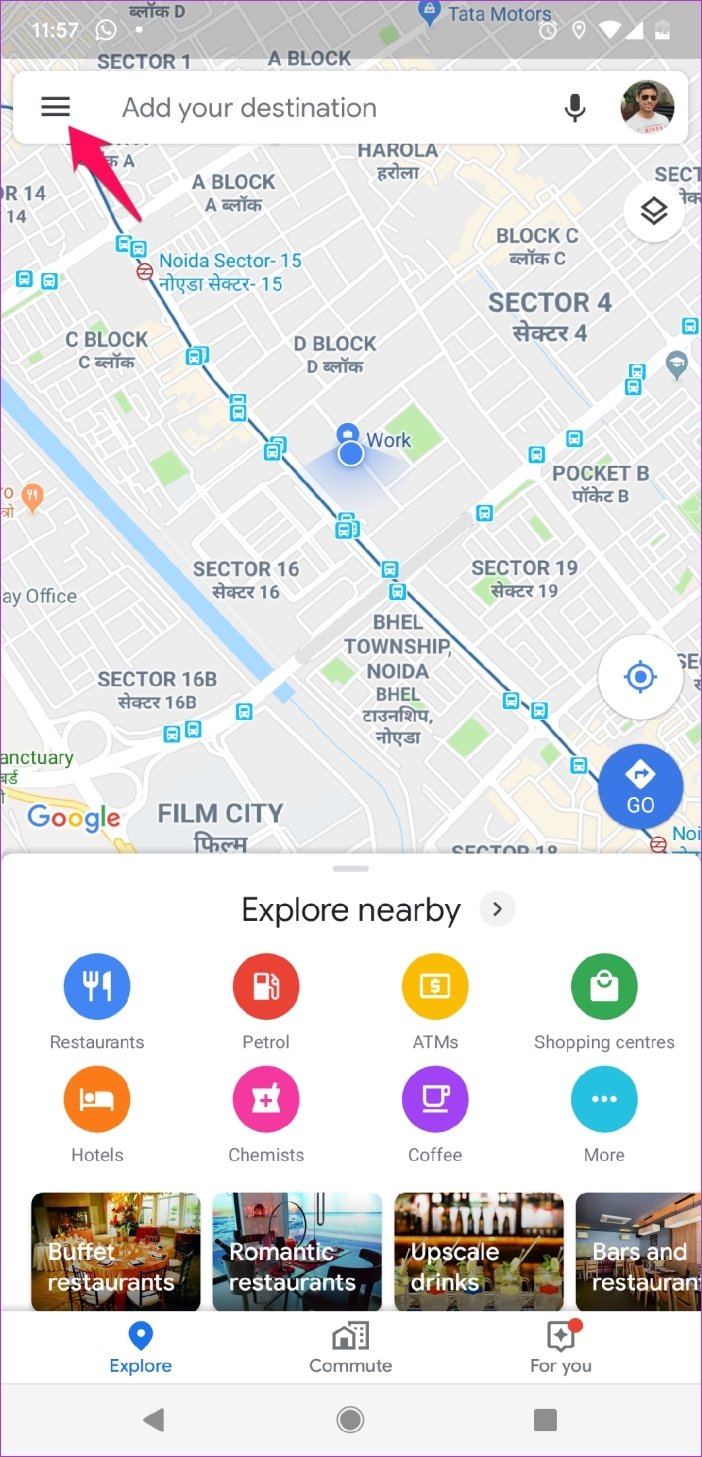The image depicts a detailed screen interface of a navigation application, likely on a smartphone. 

At the top of the screen, a status bar displays essential system information: on the left, the current time is shown as 11:57 accompanied by an alarm icon, while on the right, icons for Wi-Fi, signal strength, and battery level (approximately halfway full) are visible. Directly beneath this bar is a prompt reading "Add your destination," flanked by a tab menu indicator on the left, highlighted by a red arrow, and a microphone icon followed by a profile picture icon on the right.

Central to the screen is a map with various labels in black text. The map features a road with evenly spaced blue dots, indicating a route or points of interest, with additional dots scattered throughout. In the bottom right corner of the map is a prominent blue circle labeled "Go," and above it, a white circle with a blue dot, likely indicating the current location. 

Beneath the map, the interface offers the option to "Explore nearby," presented with eight labels in different colored circles arranged in two rows: blue, red, yellow, green on the top row, and orange, pink, purple, light blue on the bottom row. 

Further below, there are four square images representing subcategories of restaurants. The lowest section of the screen features navigational options labeled "Explore," "Commute," and "For you." At the very bottom, standard smartphone navigation buttons are present: a sideways triangle (back), a circle (home), and a square (overview) from left to right.